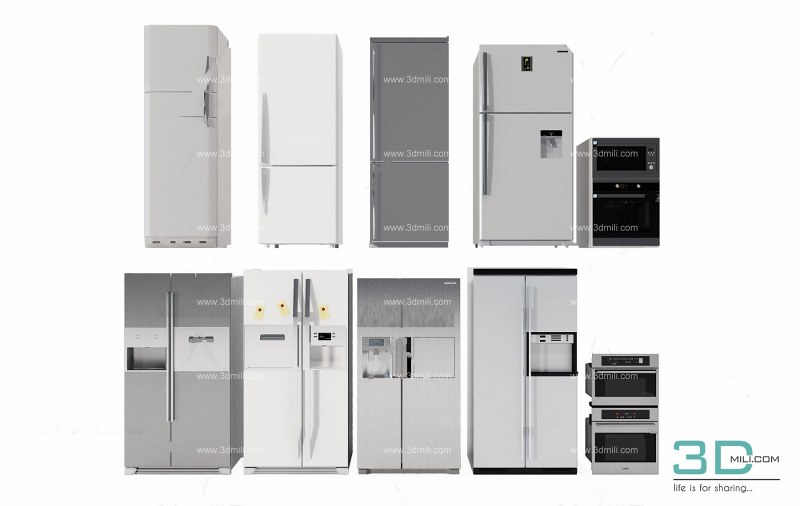The image is an advertisement showcasing a variety of refrigerators in an array of styles and configurations, set in grayscale tones of gray, white, and black. The top row features an old-fashioned slender refrigerator with a top-level freezer, a white refrigerator with a left-sided handle and larger top section, a gray refrigerator with a website www.3dmill.com printed on it, another white refrigerator with an external ice dispenser, and a mini fridge possibly designed for floor placement. The second row presents a more modern selection: a silver side-by-side door fridge, a similar model in white, followed by two silver refrigerators with external drink refill areas, and two smaller fridges stacked one on top of the other. In the lower right corner, the text "3DMillicom, life is for sharing" is prominently displayed, emphasizing the theme of evolving refrigerator designs from past to present.